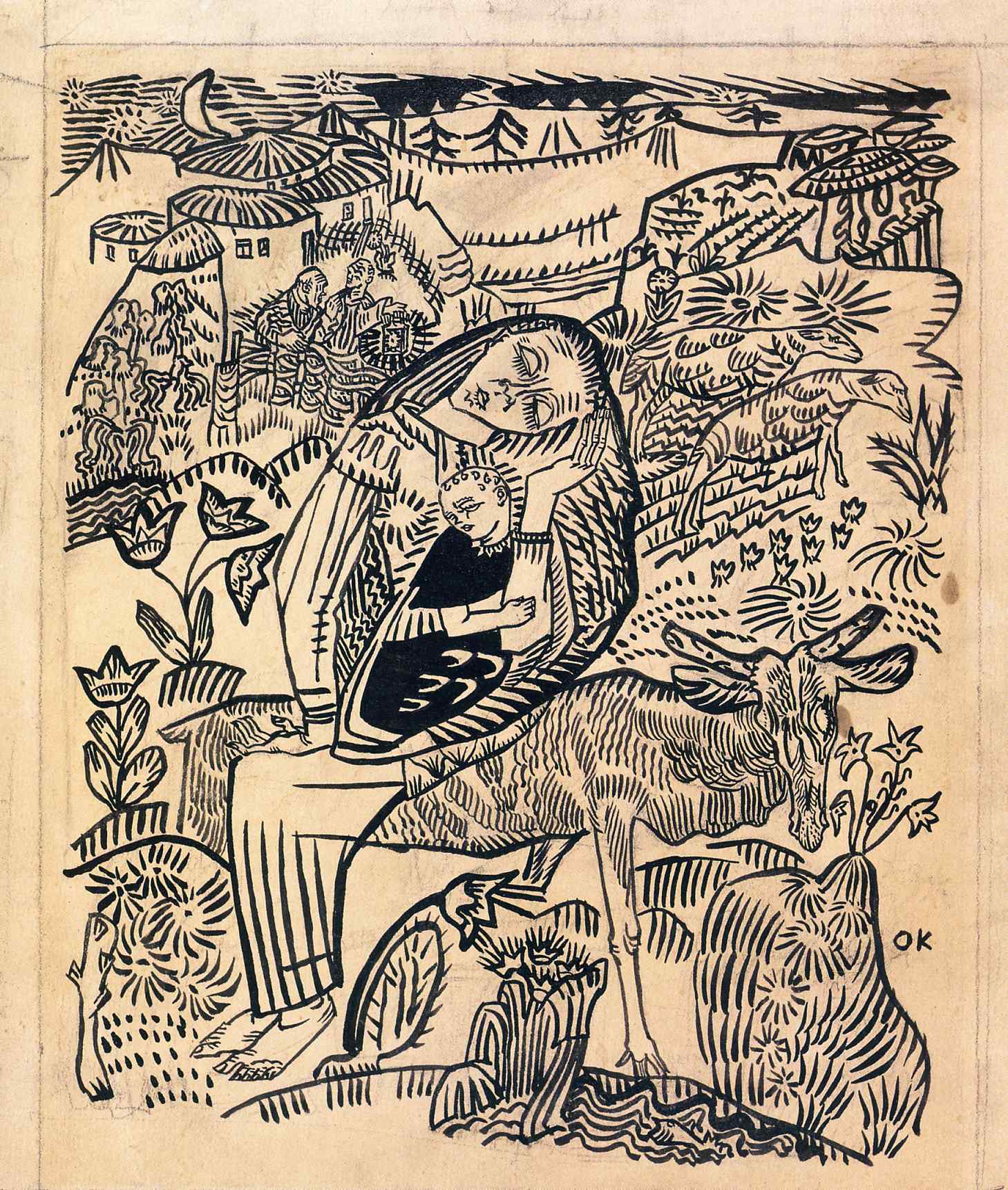This monochrome drawing, rendered in black ink on tan paper, conveys an idyllic outdoor scene with classical Madonna and Child imagery. The woman, bearing an essence that suggests she might be Mary, is depicted sitting atop a thin, horned animal—likely a deer or ram. She cradles her infant son, Jesus, who is dressed in a black outfit and gently gripping her arm. Her head is turned sideways, supported by her left hand, evoking a sense of serene contemplation. Her right hand rests lightly on her leg. Barefoot, she is adorned in a headdress that extends down to her child's position.

Two-dimensional artistic style emphasizes the figures without true perspective, creating a dreamlike quality. Around them, a detailed landscape emerges; visible flowers, plants, and rocks populate the ground. To the right of the pair, two sheep stride forward, seemingly emanating from the woman's head due to the flat plane style. In the background, a small village with thatched-roof buildings sits beneath a crescent moon, framed by distant mountains and a sky that hints at dusk or dawn. Trees and various flora are depicted above and around the central figures. A subtle text marking, "OK," is inscribed in the bottom right corner, adding an enigmatic touch to this evocative piece, reminiscent of stylistic elements that echo Picasso's sketches yet distinctly unique in its own narrative.